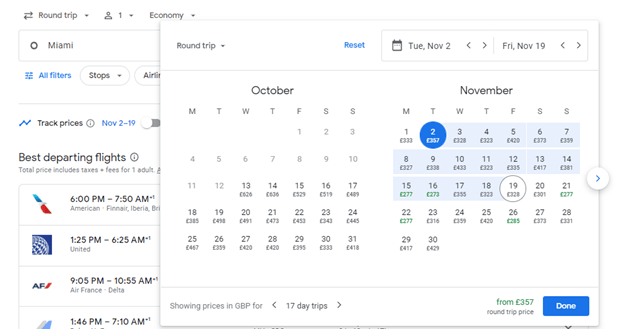Screenshot of a Flight Search Website

This detailed screenshot captures the interface of a flight search website. In the background, the main page displays a search for flights to Miami. At the top left corner, indicators show the search parameters: a round-trip flight, one passenger represented by a single person icon, and economy class selected from a drop-down menu. The city "Miami" is clearly typed into the search bar, while the filters for stops, airlines, etc., are partially obscured and not easily readable.

Overlaying the background page is a pop-up calendar for selecting travel dates in October and November. The calendar is segmented into two parts: October on the left and November on the right. Each day within the calendar displays corresponding round-trip ticket prices. Highlighted dates range from November 2nd to November 19th, with November 2nd encircled in blue and November 19th in white. This indicates the selected travel period. 

At the bottom of the pop-up, a note specifies that the prices are shown in GBP for a 17-day trip, and a round-trip price starting from €357 is prominently displayed. A "Done" button is available at the bottom right corner for finalizing the date selection.

Beneath the incomplete filters section on the main page, a list of best departing flights is shown. The top flight, with an American Airlines logo visible, departs at 6:00 p.m. and arrives at 7:50 a.m. The subsequent flight by United Airlines is from 1:25 p.m. to 6:25 a.m. An Air France (AF Airlines) flight is scheduled from 9:05 p.m. to 10:55 a.m. The final listed flight only has its times visible: 1:46 p.m. to 7:10 a.m.

Overall, the screenshot provides a comprehensive glimpse into the process of searching for and selecting flights to Miami, complete with detailed date and price information for various options.